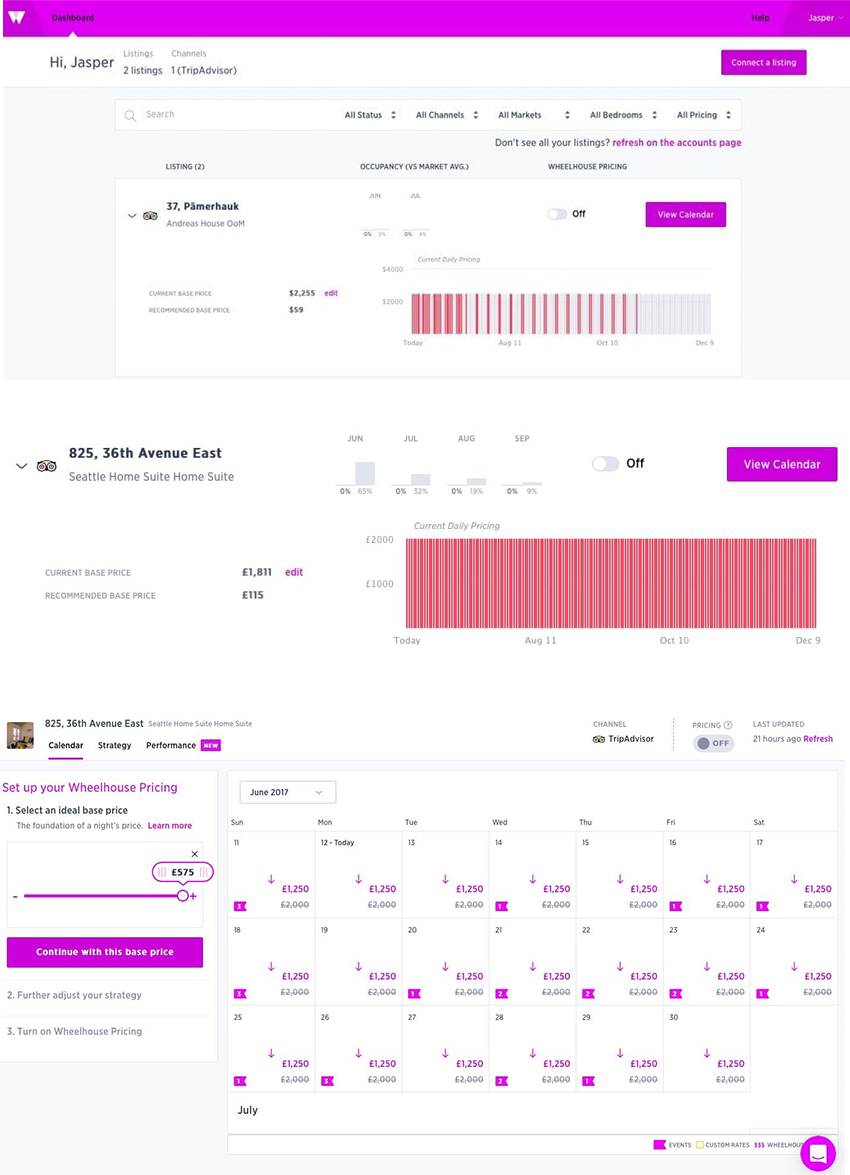This is a detailed screenshot of a management dashboard. At the top, there is a bright purple toolbar with the word "Dashboard" in black text. To the left of this, a small white icon resembling an incomplete triangle is present. On the far right of the toolbar, "Help" is displayed in black, adjacent to the user name "Jasper," suggesting it is Jasper's profile.

Beneath the toolbar, the header greets the user with "Hi Jasper" in black text on a white background. Following this are two primary listings, one of which includes a tag indicating it is a "One Trip Advisor."

The first listing is for "37 Palm Souk," seemingly referred to as "Andrea's House." This section includes a small barcode-like graphic in grey and red and offers an option to view the calendar, though the specific purpose of this listing (whether for selling or renting) is unclear.

The second listing is for "825 36th Avenue East, Seattle Homesuit Homesuit," featuring a barcode in red with evenly spaced lines. This barcode, similar to the first listing, displays a price and dates.

At the bottom of the dashboard, there is a calendar for June 2017, which shows various prices marked in purple and grey.